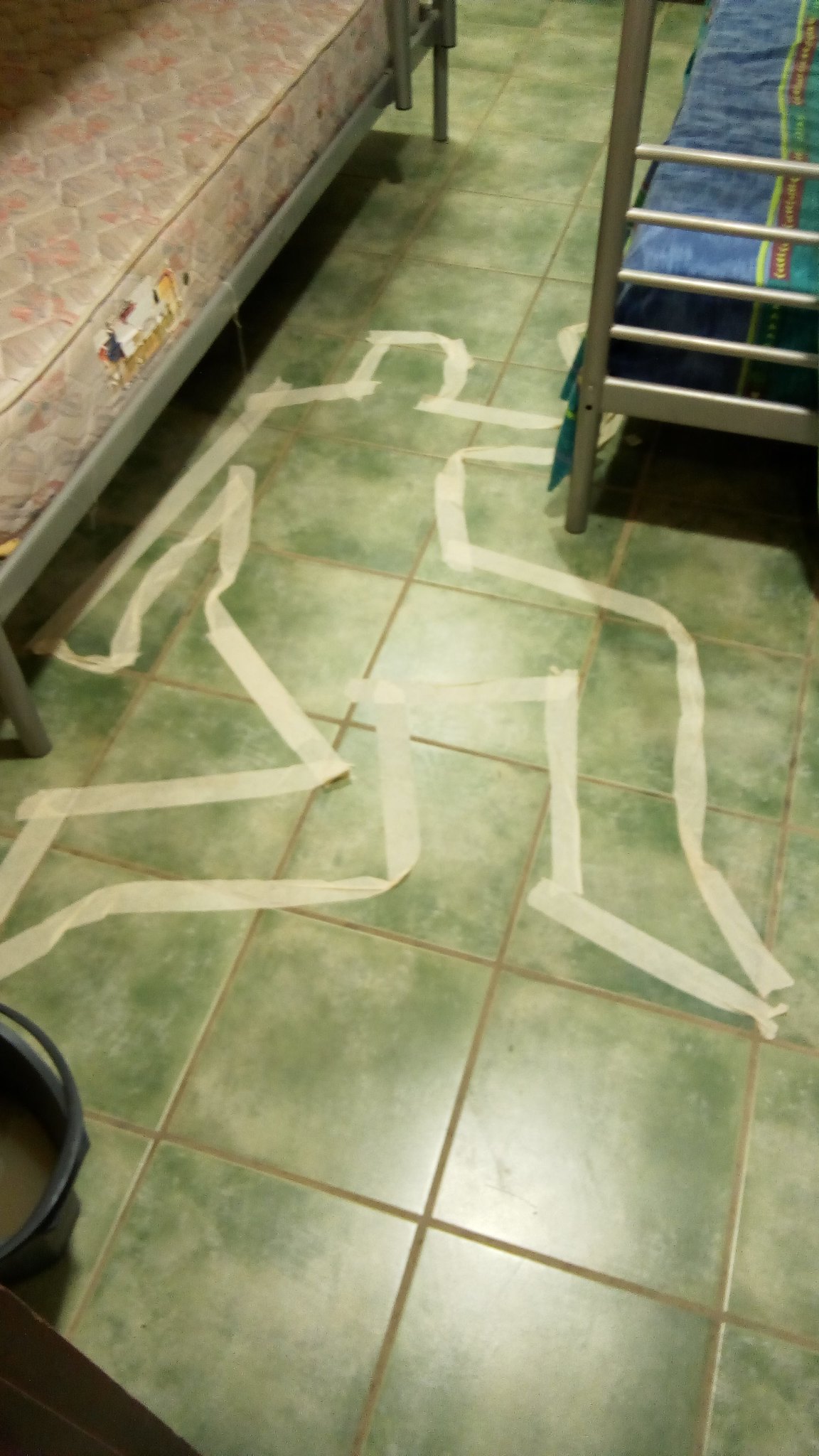This photograph depicts a scene from above, focusing primarily on a crude outline of a body formed with white masking tape on the floor. The floor consists of large, ceramic green and white tile squares that give a cloud-like pattern. The outline, resembling where a body once laid, is placed humorously or mock-seriously between two metal-framed beds, suggesting a prank rather than a genuine crime scene, due to the lack of police tape and the informal appearance. 

To the left of the tape outline, there's a mattress with a floral pink pattern, while the bed to the right features a blue, yellow, and red striped blanket. Both beds appear to be simple dormitory or barrack-style twin beds, accentuating the starkness of the scene. The tape outlining the body is somewhat haphazardly applied, with one arm depicted as straight down by the side and the other bent upwards. The imagery, especially with the beds' positioning and the crude tape outline, evokes a sense of staged dramatics in an otherwise mundane setting.